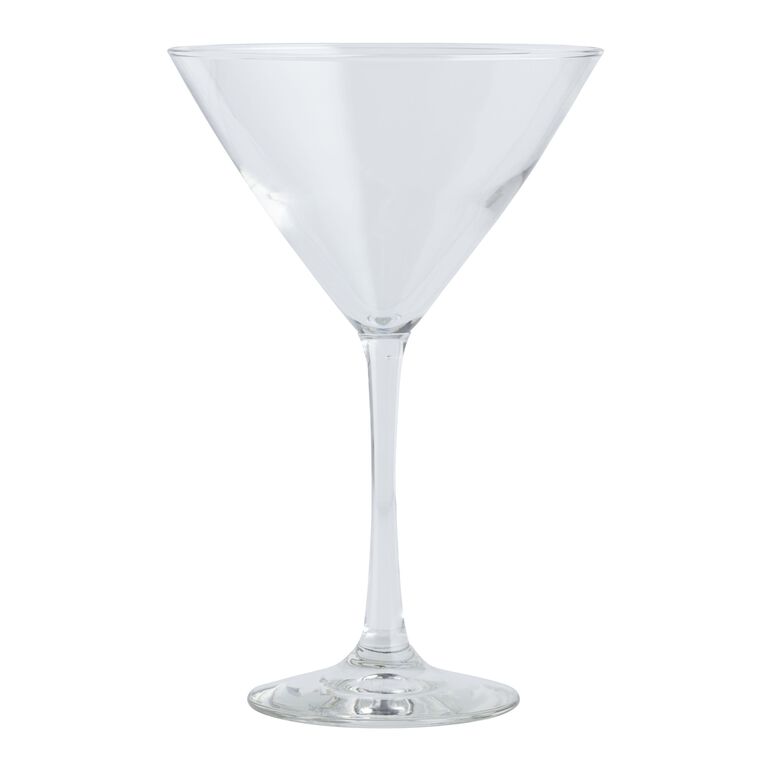The image displays a cocktail glass, likely a martini or margarita glass, set against a plain white background. The glass features a round base that transitions into a long, slender stem. This stem supports the upper portion of the glass, which is shaped like an inverted cone or funnel and flares out widely at the top. The top part of the glass appears frosted, rendering it opaque, while the bottom portion is transparent. The glass is centrally positioned within the image, which contains no text or additional elements.